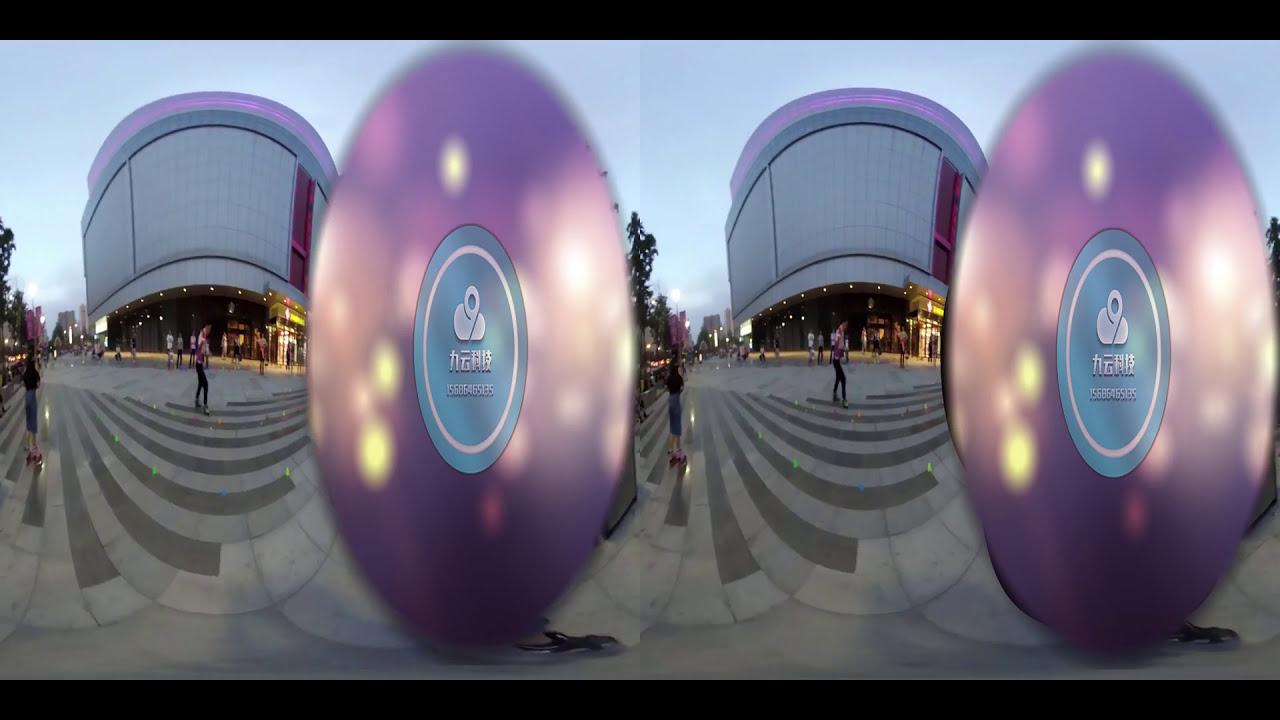The image depicts a bustling cityscape featuring a large, modern building that resembles a shopping mall or arena. The scene is captured in an urban environment during dusk or near sundown, as evidenced by the illuminated streetlights. The building is characterized by its substantial size, with white, circular architecture and an abundance of lights, contributing to an inviting ambience. The exterior is composed of gray tiles and concrete panels, and the entrance on the right side is marked by yellow text above the doorway.

The city square in front of the building features light gray and dark gray lines crisscrossing the ground, with several pedestrians, who appear to be Asian and dressed up, walking purposefully through the scene. The background architecture suggests a lively, metropolitan area.

A peculiar aspect of the image is its duplicated nature, split vertically down the middle, creating mirrored visuals on the left and right sides, similar to the effect seen in 360° videos. Furthermore, a large, oval-shaped blob covers a significant portion of the right side of the image. This blob is predominantly purple with a blue inner circle outlined in white. It includes a pin icon on a cloud and white Chinese text, hinting at some kind of digital interface or augmented reality element within the photograph.

Overall, the image conveys a dynamic and contemporary urban scene, highlighted by both physical and digital overlay elements.